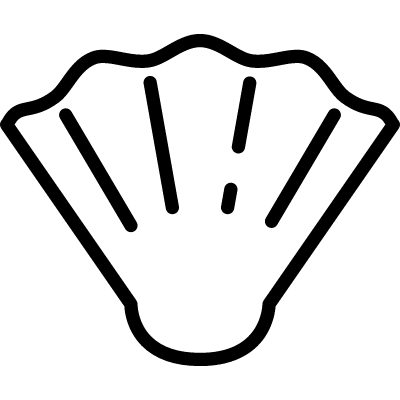The image is an artistic, black-and-white outline that mimics a seashell or possibly a flipper, characterized by a highly symmetrical, wavy edge at the top. The bottom of the outline is rounded, and it fans out towards the sides in a V-shape, further emphasized by the wavy top. Within the shell-like design, four vertical black lines run through the middle against a white background. The third line from the left is distinctively broken, with a gap of white space before it continues, adding a subtle imperfection to the otherwise methodical pattern. The black outline and lines are of medium thickness, giving the image a clean and exact appearance.